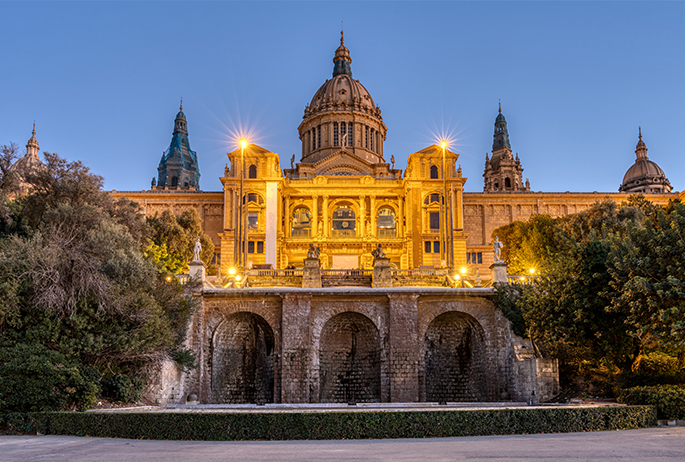This image captures the majestic front of a large, historic European architectural building, likely situated in an old European city. The building, resembling a grand castle, palace, or possibly a government structure like a Capitol Hall, is constructed from grayish brick or rock, exuding an aged elegance. Prominent among its features are the towers; there are five in total, with two rectangular towers flanking the entrance and three larger towers—two with pointy tops and one central tower crowned with a circular dome. The building also boasts multiple domes and several statues of people adorning the facade. The front entrance is marked by three archways, leading into the expansive structure. Surrounding the entrance are trees on both sides and a notable fountain in the foreground. The structure is illuminated by bright lights, suggesting the photo was taken in the evening as the sky transitions to dusk, revealing a clear, darkening backdrop. With intricate stained glass windows and a welcoming parking lot, this architectural marvel stands as a testament to its historical and aesthetic significance, inviting onlookers to explore its grandeur.